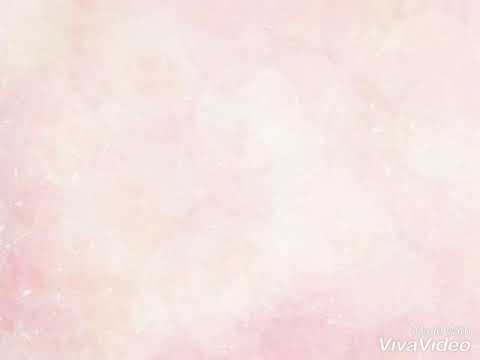This image is a small rectangle, approximately three inches wide and two inches high, featuring a dreamy, abstract background composed of various shades of pink, peach, off-white, and faint gray. The colors are blended smoothly, resembling a soft, cloud-like mix or a delicate pink overlay with some lighter white areas showing through. The center of the image is slightly brighter and whiter compared to the edges, enhancing the overall ethereal effect. In the lower right-hand corner, there is faint gray text divided into two lines. The top line is illegible, while the bottom line clearly reads "Viva Video," with both "V" letters capitalized. The image lacks any distinct borders, headers, or footers, maintaining a seamless and borderless appearance.